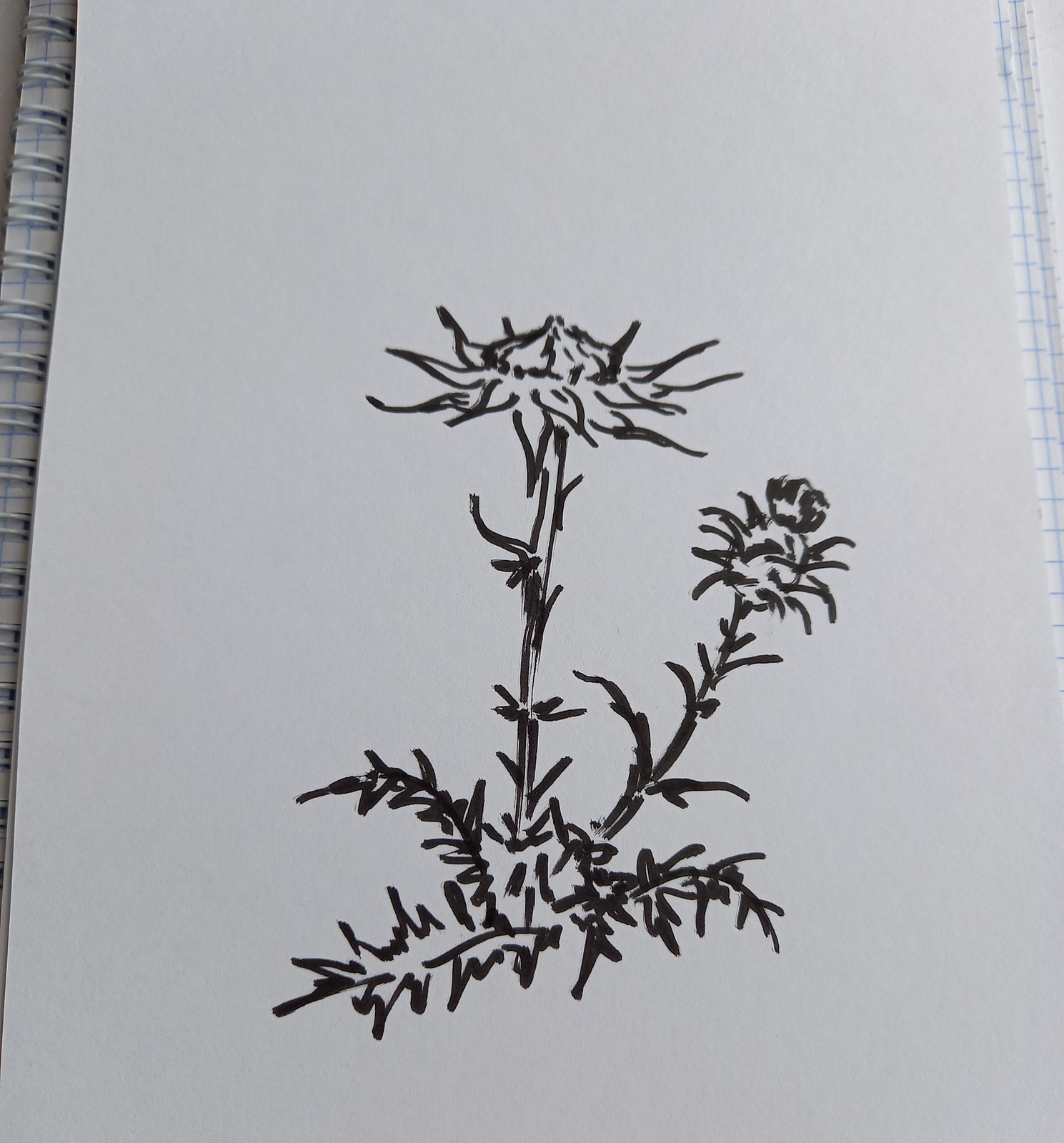The image is a detailed pen drawing, possibly using Japanese calligraphy ink for its style, done on white stock paper that sits atop a notebook, with visible binding on the left side. The notebook underneath is graphing paper, identifiable by the hint of blue lines and the spiral binding. The sketch depicts two thistle stalks, each crowned with a flower; the left flower bud is fully open and the larger of the two, while the right one is partially open. The drawing conveys a sense of simplicity yet artistic finesse, with spiny leaves clustering at the base of the stalks and some extending partway up. The overall stark black strokes against the white backdrop emphasize the spiky, intricate details of the thistle flowers and their stems.